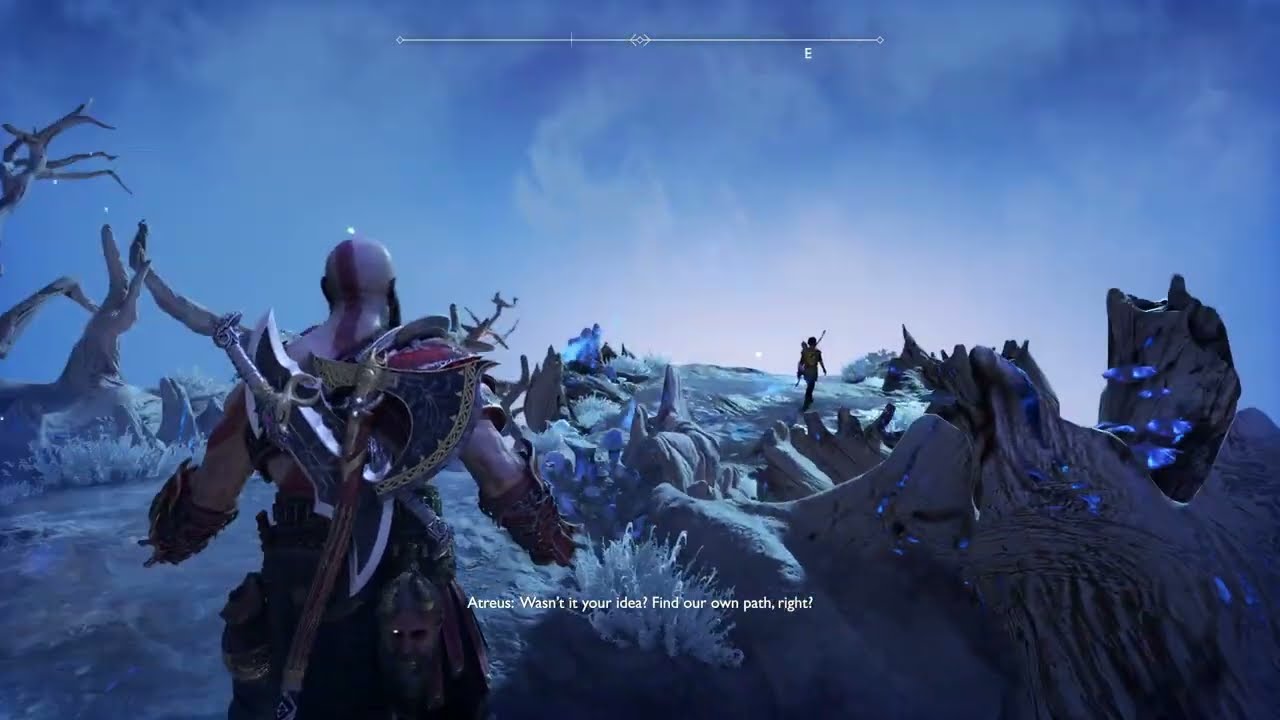The image displays a screenshot from a third-person video game set in an icy, desolate environment dominated by varying shades of blue. The scene is horizontally rectangular with a gradient sky, transitioning from dark to lighter blue towards the center, interspersed with faint wisps of blue clouds. The ground mirrors this blue-gray palette, featuring barren, broken trees and scattered grayish-blue rocks and shrubs. 

In the foreground, just left of the center, stands a very muscular, bald character with a prominent red stripe running from the center of his head down his back. This warrior is equipped with a large battle axe, a sword, and wears sizable gauntlets, though the backs of his elbows are exposed. Notably, there is a severed head attached to his belt. The white text overlaying the scene reads, "Atreus, wasn't it your idea? Find your own path, right?" In the background, another character is seen walking away from the main figure, contributing to the scene's narrative and adding depth to the landscape.